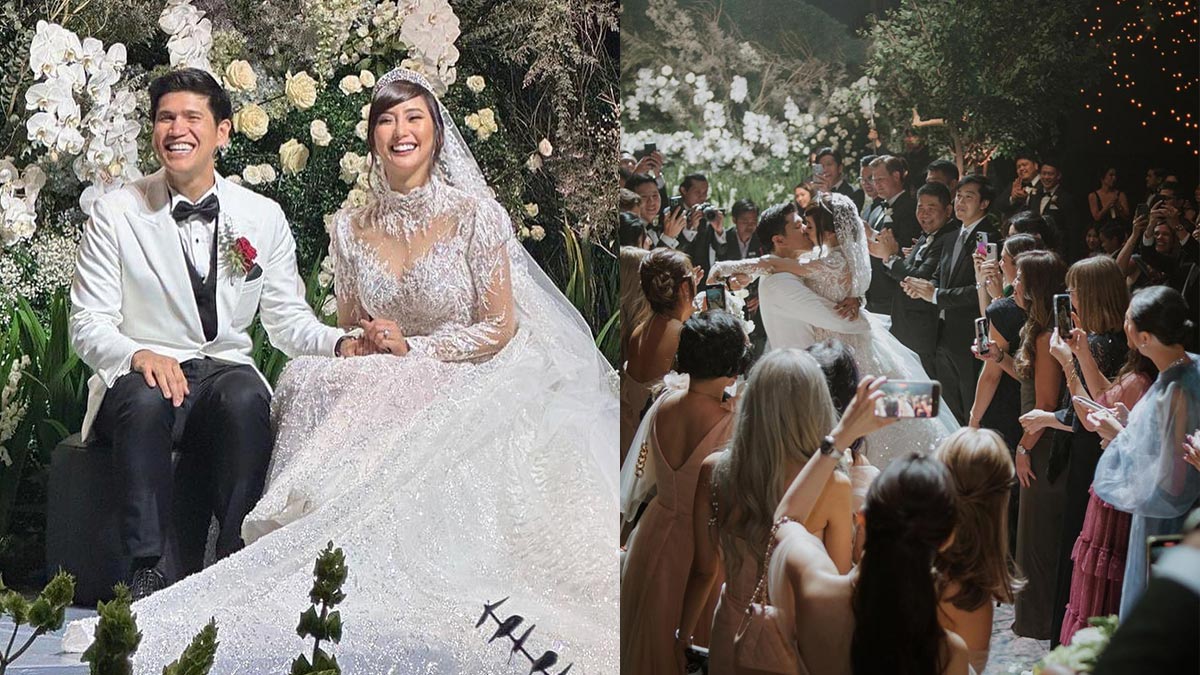This image features two photos side by side capturing moments from a wedding. In the left photo, the groom, who has dark hair, is smiling and dressed in a white tuxedo jacket with black pants, a black bow tie, and a red rose on his left lapel. He stands beside his bride, who has brown hair and wears an ornate white wedding gown with a lace veil. Behind them, a green shrub adorned with white roses creates a picturesque backdrop.

In the right photo, the groom is seen lifting and kissing his bride amidst a joyful crowd. The guests, dressed in suits and elegant attire, form a celebratory circle around the couple. The setting includes lush greenery, with small lit lanterns and a tree enhancing the festive atmosphere. The bride and groom's embrace captures the joyous spirit of the event, surrounded by friends and family.